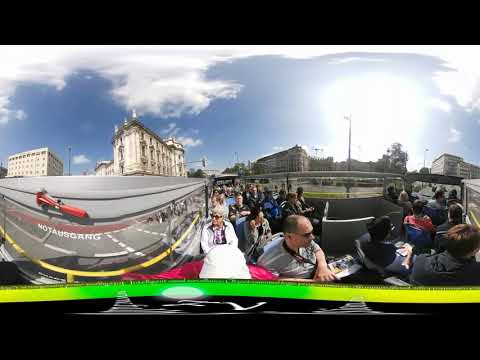This panoramic photograph captures a vibrant and busy scene of people seated on a roofless tour bus during a sunny day in a city. The bus is filled to capacity, with two rows of seats separated by a central aisle, and all the seats occupied. The image presents a dynamic view from the top of the bus, where people are funneled through a narrow section, leading to stairs that descend towards the back.

In the background, the cityscape features an array of tall, old buildings, with one strikingly oblong structure adorned with a green roof. Adjacent to it stands a pristine white office building characterized by numerous windows. A tall lamppost can be spotted between these buildings.

The upper portion of the image reveals a blue sky accented with white clouds, which are more prominent on the left side of the frame. The sun shines brightly from the upper right corner, casting a glow that enhances the atmospheric perspective. The lower portion of the photo includes a black border with a yellow and green wave-like graphic that is somewhat obscured by a circular sun emblem and white text that is not completely legible, possibly indicative of the bus's branding or route information. This layered visual composition offers a detailed snapshot of a bustling urban adventure.